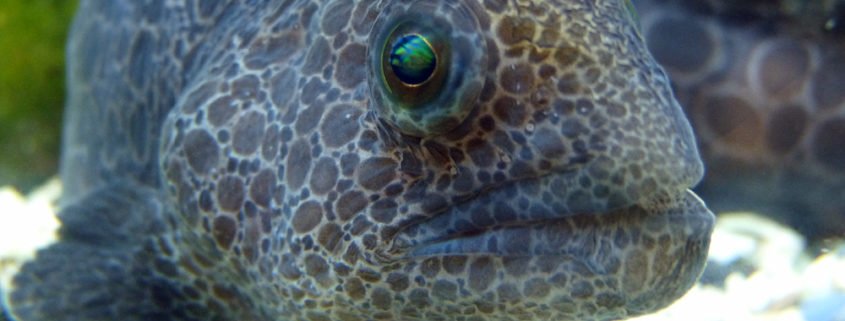This realistic and very close-up image likely depicts an underwater creature, possibly a fish or an eel, displayed prominently in a wide, horizontal rectangle. The focal point is a bright green, metallic sheen eye positioned at the very middle of the image, which peers slightly to the right. Surrounding the eye, the creature's skin features a complex texture: light tan lines interwoven in a circular grid pattern, interspersed with large dark brown splotches, giving it a camouflage-like appearance akin to rocks on tan sand. The fish's head, slightly blurry, shows a closed mouth and the illusion of movement as if photographed through aquarium glass, suggested by the cyan tint and blurred greenery in the background. The body extends off to the left, curving back to form an S-like shape, adding to the impression of it being coiled within an underwater habitat. The presence of reflected green and blue hues adds a sense of depth and realism to the aquatic scene.